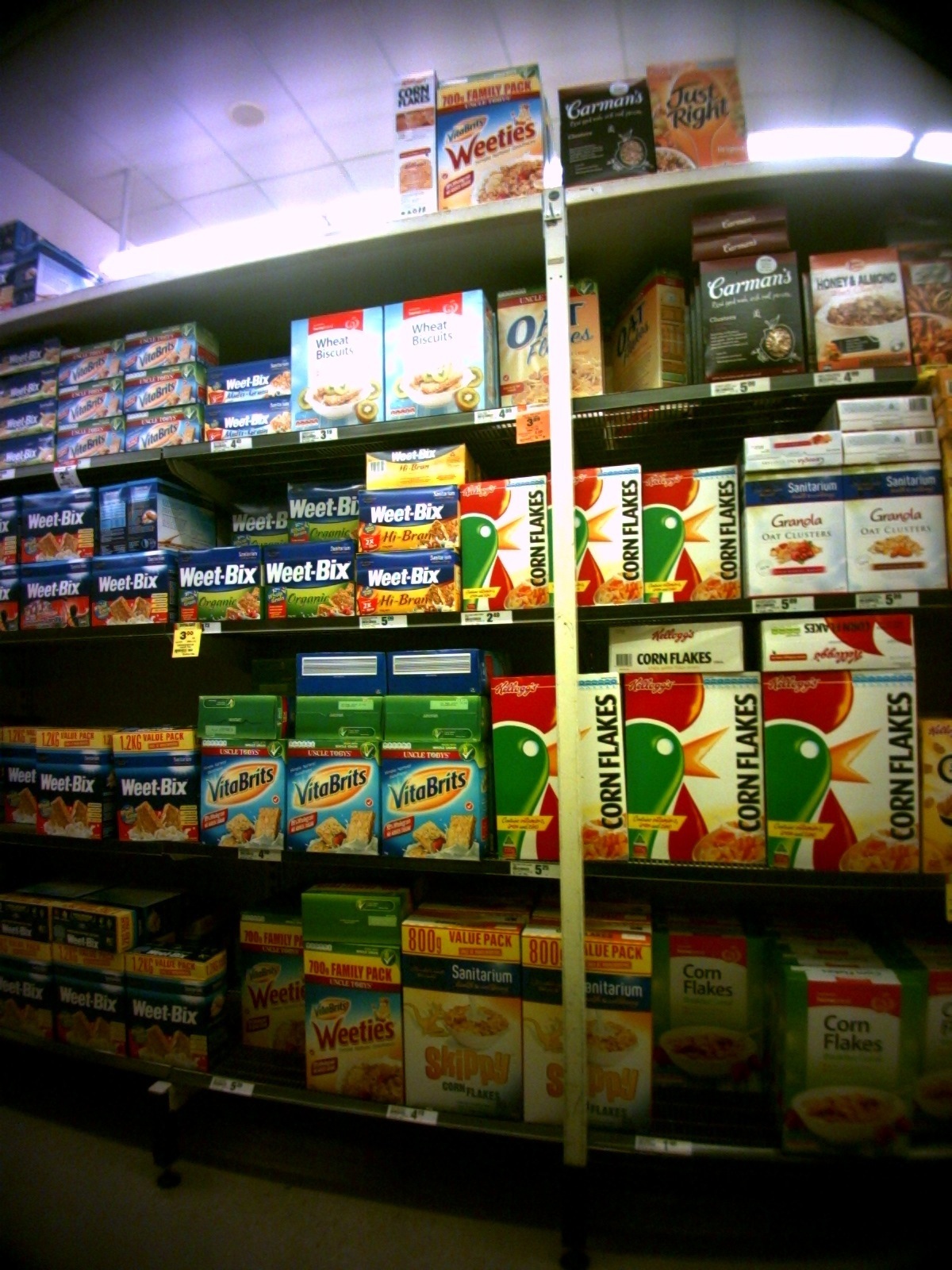This photograph captures a grocery store aisle lined with a shelf stocking various cereals. The shelving unit has five horizontal tiers filled with different cereal boxes. The top shelf prominently features large boxes of Corn Flakes, Wheaties, Carmins, and Just Right. The second shelf displays additional varieties of Corn Flakes, Wheat Bix, and Vitabrits. The lower shelves include brands such as Skippies and more boxes of Corn Flakes and Wheat Bix. The floor beneath is a greenish-gray hue, while the white ceiling above is fitted with fluorescent lighting. The image has a low resolution, making some of the lettering on the cereal boxes difficult to discern, but the organized layout of the cereal boxes and the price tags on the shelves are still recognizable.